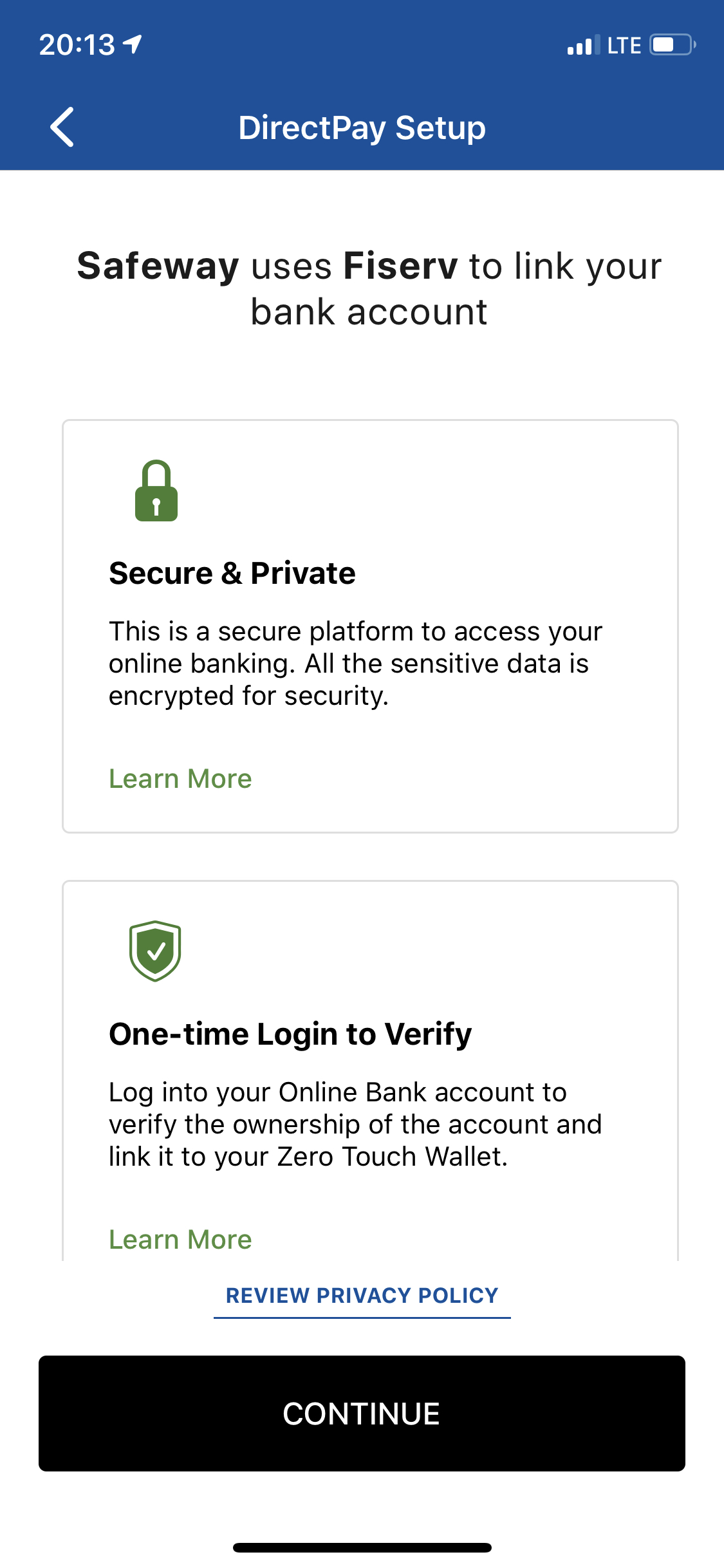Screenshot Description: Secure Direct Pay Setup on a Banking App Interface

The image is a screenshot of a mobile phone displaying the Direct Pay setup screen within a banking app. The screen is sectioned with a blue banner at the top, indicating the step for setting up Direct Pay. Below the banner, on a white background, it states that "Safeway uses Fiserv" (spelled out as F-I-S-E-R-V) to facilitate linking your bank account.

The interface features two informational sections, both highlighted with icons to emphasize security:
1. **Secure and Private**: Marked by a padlock icon, this section assures users that the platform is secure and encrypted, ensuring the safety of sensitive data. There is also a green "Learn More" link available for users who seek additional information.
2. **One Time Login to Verify**: Accompanied by a shield icon with a checkmark, this section instructs users to log in to their online banking account. This one-time login is required to verify account ownership and link the bank account to the ZeroTouch wallet. Additionally, there are options to "Learn More" and to review the "Privacy Policy" via a blue link.

At the bottom of the screen, there is a prominent black "Continue" button which users can tap to proceed with the Direct Pay setup.

The overall layout and details suggest that the app focuses on security and privacy for bank account linkage and potentially utilizes a feature or service named ZeroTouch wallet within its system.